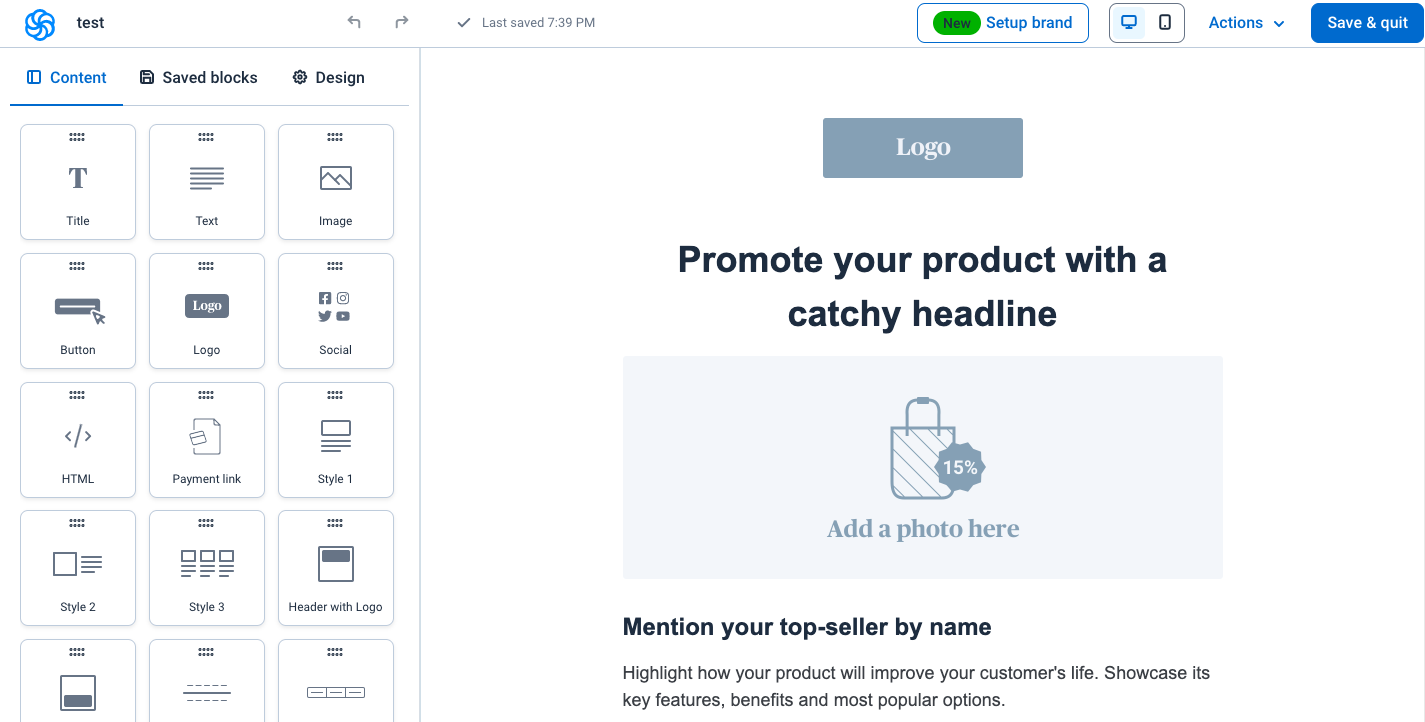This screenshot, taken in landscape mode, captures a detailed user interface of a website design or content management tool. The interface is divided into two columns:

**Upper Left Section**:
- Exhibits status information with the initial text displaying "test."
- Subsequently switches to indicate "last save: 7:39 p.m."
- Features a blue "Clear" button with the label "Set up brand."
- An adjacent green circle labeled "New."

**Top Controls**:
- A button to toggle the view between landscape and another mode.
- An "Actions" button with a dropdown menu.
- A blue "Save and quit" button.

**Left Column**:
- A vertical tab menu highlighted with the following options:
  - *Content* (highlighted in blue and underlined)
  - Save Blocks
  - Design
- Various content elements listed under the Content tab, including:
  - Title
  - Text
  - Image
  - Button
  - Logo
  - Social
  - HTML
  - Payment Link
  - Styles (Style One, Style Two, Style Three)
  - Header with Logo

**Central Column**:
- Display area with an initial placeholder logo and a logo upload button.
- A headline section prompting the user to "Promote your product with a catchy headline."
- A large gray area with the text “Add photo here.”
- Text instructions for further content: "Fifteen percent. Mention your top seller by name. Highlight how your product will improve your customer's life. Showcase its key features, benefits, and most popular options."

This comprehensive layout provides a convenient platform for users to arrange their website’s content, customizing it through various tabs and content elements.